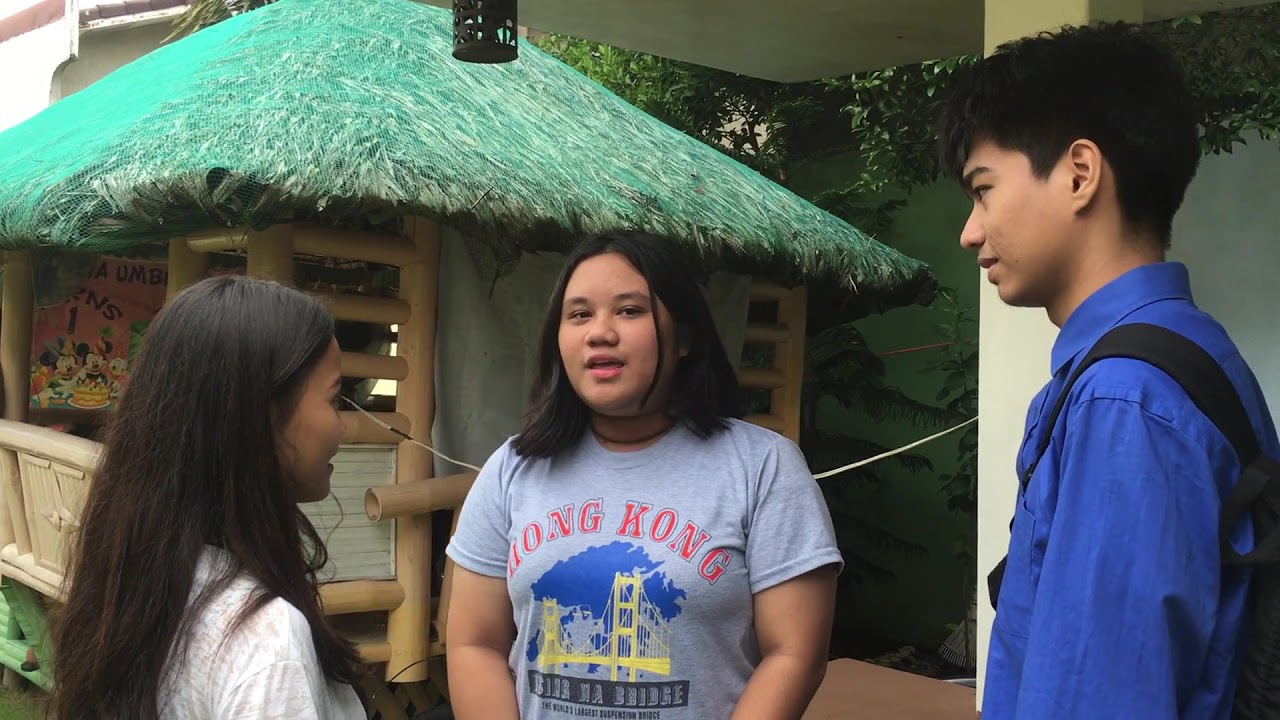This full-color photograph, taken outdoors on a sunny day, captures three teens engaged in a moment of interaction against a backdrop of trees and an artificial grass hut that resembles a souvenir shop, possibly featuring Disney characters like Mickey Mouse. The image is horizontally rectangular, measuring about six by three inches.

The tallest of the three, a boy, stands on the right. He has dark black hair cut neatly around his ears and neck and wears a long-sleeved blue button-up shirt with a black backpack strap over his shoulder. He gazes towards the girl in the center.

The central figure is a girl with straight black hair parted in the middle and shoulder-length. She has brown skin and wears a gray t-shirt with "Hong Kong" written across it in red, adorned with an image of a bridge. She is looking slightly off to the side of the camera, her mouth open as if speaking.

To the left stands another girl with long dark brown hair, only partially visible as she faces the boy. She wears a white shirt and engages in conversation with her companions. Behind them, the lush trees frame the scene, adding to the natural outdoor ambiance.